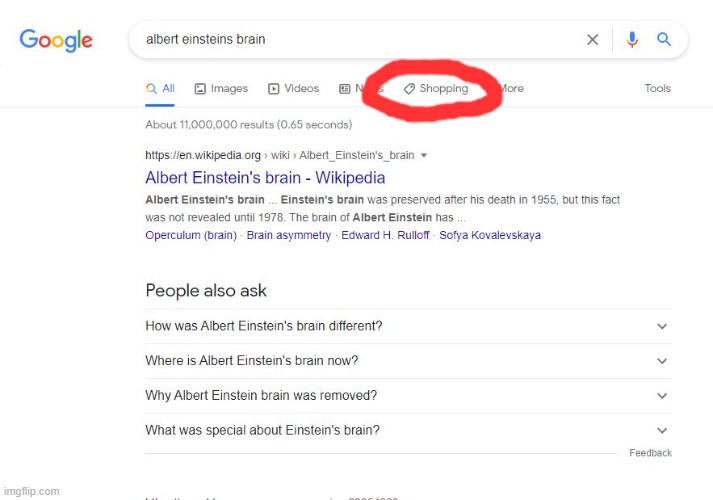This image is a detailed screenshot of a Google search results page with a clean, white background. In the upper left corner, the iconic Google logo is prominently displayed, featuring the letters "Google" in the signature colors: blue G, red O, yellow O, blue G, green L, and red E. The search query entered, "Albert Einstein's brain," is clearly visible in the search box at the top of the page.

Directly beneath the search box, the navigation tabs span from left to right, starting with "All," followed by "Images," "Videos," "News," and "Shopping." The "Shopping" tab stands out, as it is encircled by a conspicuous, hand-drawn red circle. To the right of "Shopping," additional options "More" and "Tools" are visible.

The first search result prominently featured is from Wikipedia, titled "Albert Einstein's brain - Wikipedia." The snippet under this result briefly details that Einstein's brain was preserved post-mortem in 1955, though this fact remained unknown until 1978. The snippet intriguingly cuts off mid-sentence, with "The brain of Albert Einstein has..."

Below the first result, a "People also ask" section is visible. This section lists several frequently asked questions about Einstein's brain, each accompanied by a downward arrow indicating a dropdown menu for more information. The questions include: "How was Albert Einstein's brain different?" "Where is Albert Einstein's brain now?" "Why was Albert Einstein's brain removed?" and "What was special about Einstein's brain?" 

The screenshot provides a succinct overview of Google search results for anyone inquiring about Albert Einstein's brain, including additional resources and related questions for further exploration.